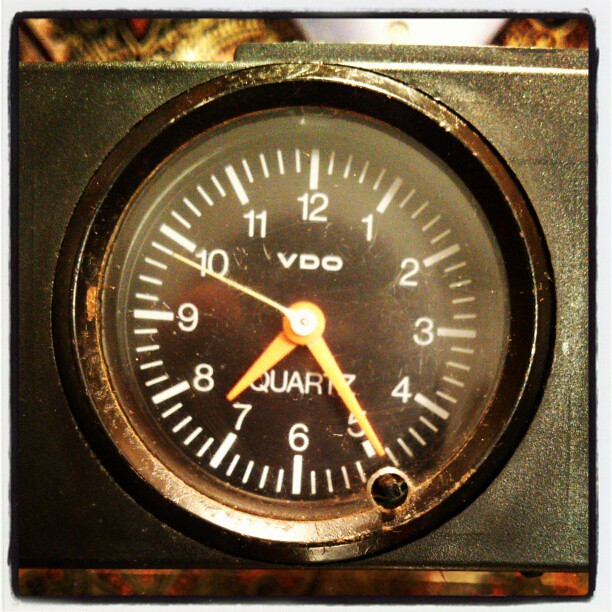This close-up photograph features a small clock reminiscent of those found on vehicles or motorcycles, evoking the appearance of a gauge. The clock has a distinctive square shape with a circular face set within the square frame. The frame is constructed from a black material, while the circular face is outlined in black metal, adding a touch of contrast. The background of the clock face is black, with white notches, numbers, and letters providing clear readability.

At the top, beneath the number 12, the letters "VDO" are prominently displayed. The word "quartz" is positioned above the numbers 7, 6, and 5, indicating the clock's mechanism. The clock hands are boldly colored for visibility: the hour and minute hands are a vibrant orange, and the second hand is a striking white. The clock indicates the time as 7:25, with the second hand poised just before the number 10 notch.